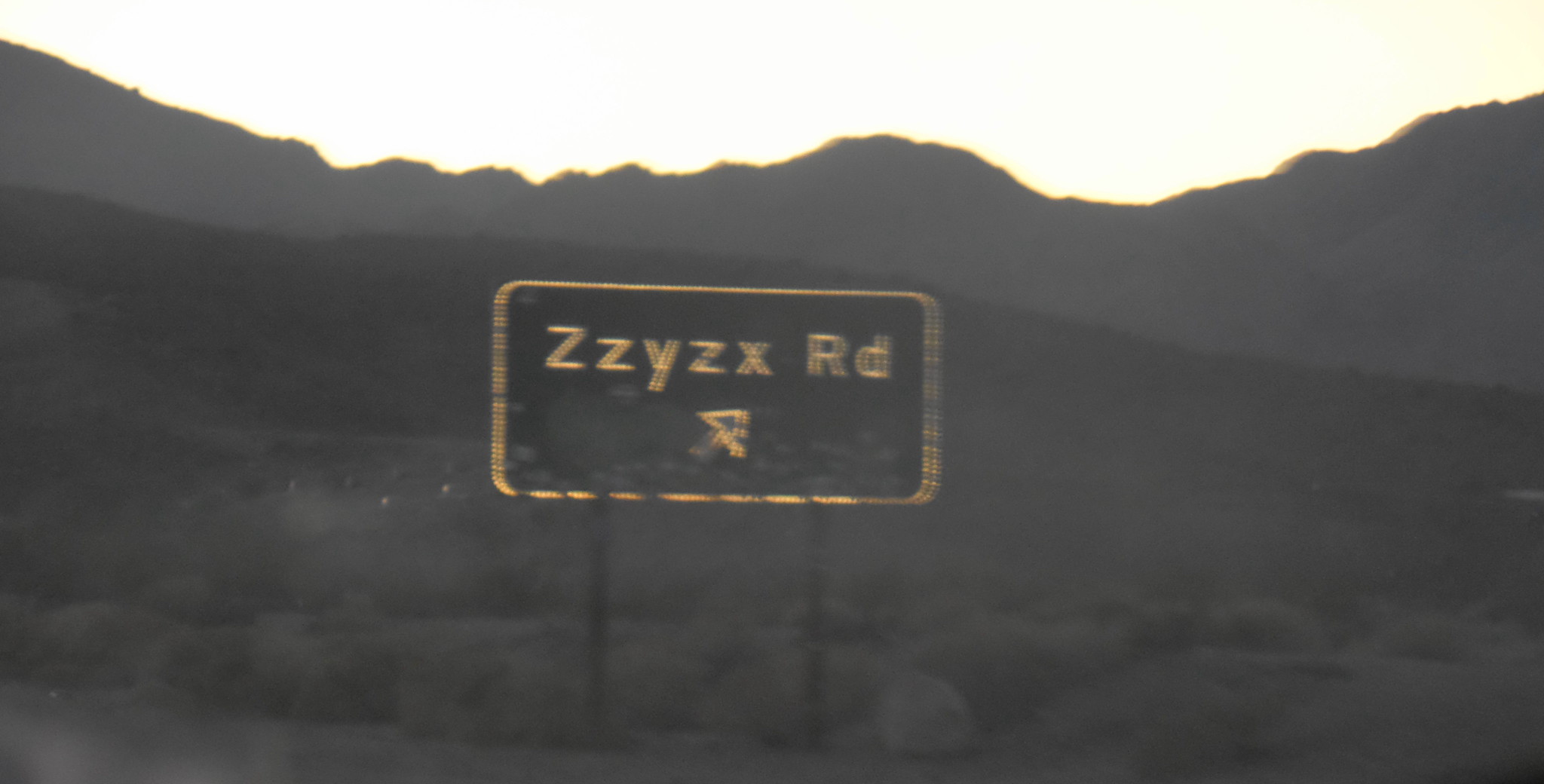This close-up black and white photograph, seemingly taken during early morning or late evening, captures a stark desert landscape. Central to the image is a street sign with the text "ZZYZX RD" in white, set against a black background with a white-bordered arrow pointing northeast. The reflective-edged sign stands amidst a mix of bare land and scattered short, greyish plants, possibly sagebrush. A vast, dark grey mountain range ascends from left to right in the background, under a grey sky subtly illuminated by a faint white-yellowish light, suggesting the time of day to be around dusk or dawn.